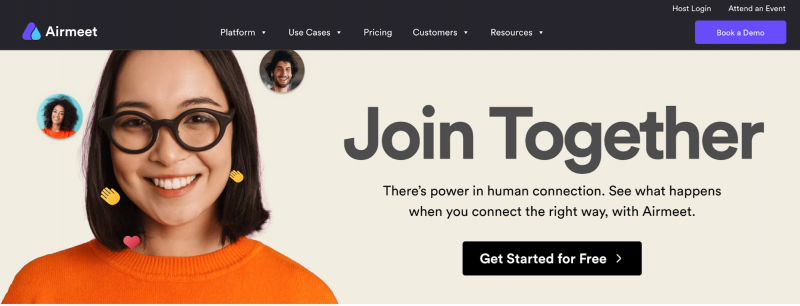The screenshot showcases the top portion of a website or app interface, believed to be associated with Airmeet. The design begins with a black navigation bar at the very top, featuring a white "Airmeet" text on the left side, accompanied by a distinctive purple and green logo representing the brand's visual identity.

Centrally positioned within the black border are several drop-down menu options labeled "Platform," "Use Cases," "Pricing," "Customers," and "Resources," all in white font. To the far right is a prominent button labeled "Book a Demo," also in white. Above this button, there are links for "Host Login" and "Attend an Event" in smaller white font.

Beneath the navigation bar, the hero section of the page is displayed. It features a large background image with a beige hue. In the foreground, on the left side of the image, there is a smiling woman with glasses, dressed in a sporty style with large dangly earrings and an orange shirt. Surrounding her are two smaller circular profile images.

The hero text, prominently displayed in large font, reads: "Join together. There's power in human connection. See what happens when you connect the right way with Airmeet." Following this text is a noticeable "Get Started for Free" button, inviting users to engage further with the platform. This screenshot represents the top section of the website, providing a glimpse into Airmeet’s user interface and branding strategy.